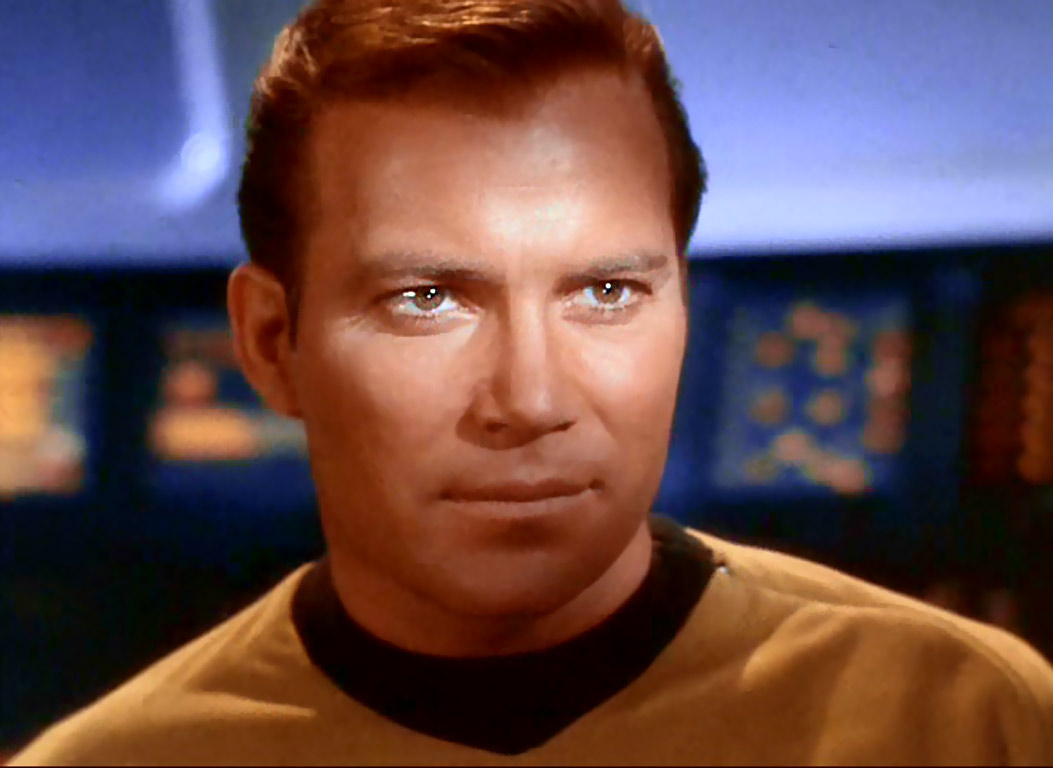The image captures a young William Shatner portraying Captain James T. Kirk from the 1960s television sci-fi series, Star Trek. He is seen in his iconic mustard captain's shirt with a black collar. His short, styled brown hair shines under the studio lights, highlighting the meticulous attention to detail in his appearance. A strip of light draws focus to his expressive light brown eyes as he gazes intently off-camera. The background indicates he's aboard the starship, featuring a blue panel with several orange dots and bars, although specific details are obscured by Captain Kirk's broad shoulders. A panel to his right and another to the left of his head are richly hued in orange, contributing to the authentic set design that immerses the viewer in the Star Trek universe.